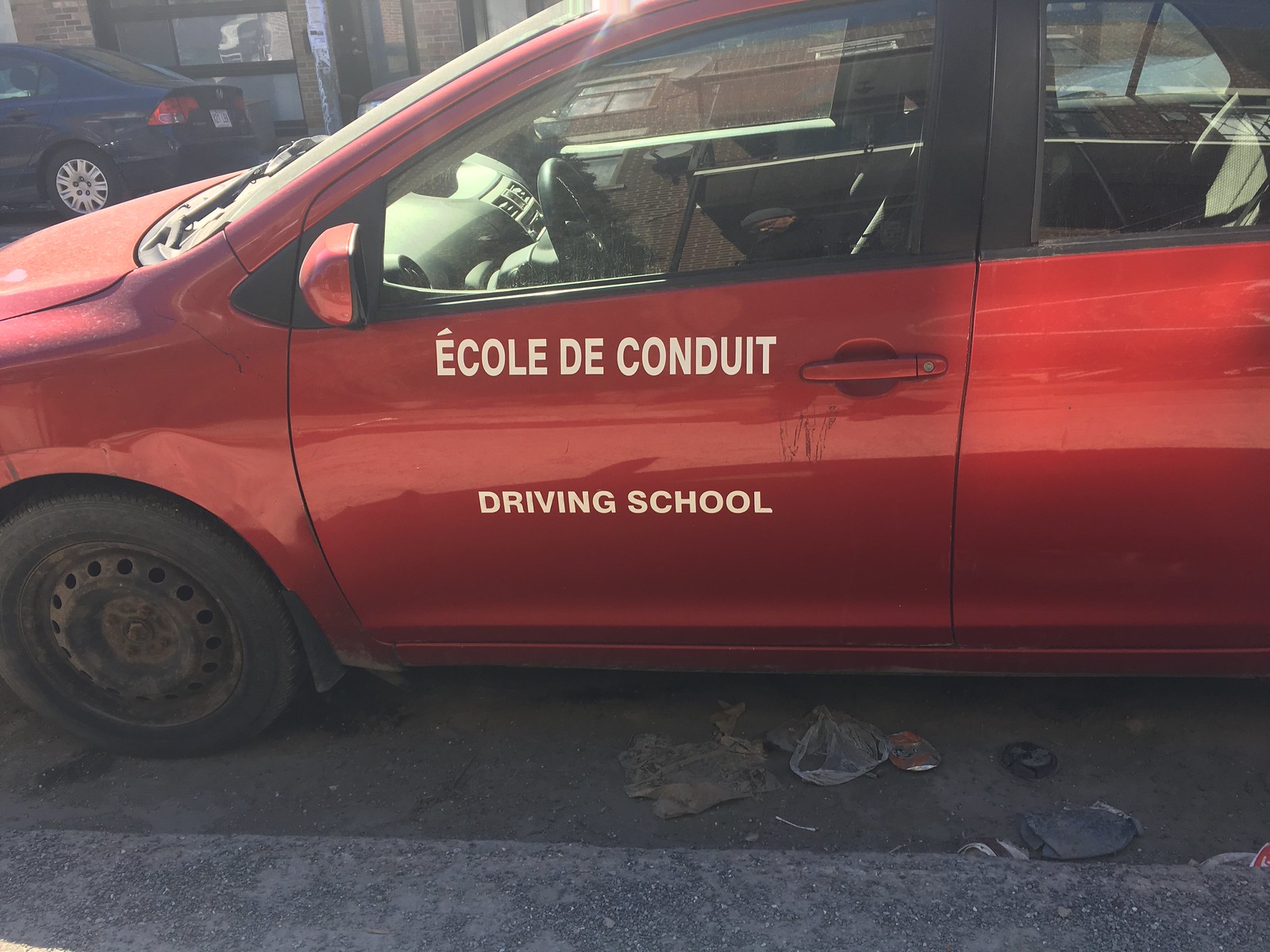The image depicts a red, somewhat old and worn car, clearly used for driver's education, as indicated by the words "Ecole de Conduit" and "Driving School" inscribed in white on its side. The car's front left tire is dirty and appears corroded, with no hubcap and significant signs of wear. Notably, there seems to be scratches around the door handle and potentially a dent on the front right fender. The vehicle is parked beside a curb, with a noticeable accumulation of garbage underneath, including plastic bags, crushed cans, and other trash. In the background, towards the right, the rear end and back left tire of a black car are visible, positioned in front of a building with glass windows. Across the street, there’s a blue car, which appears to be in better condition, parked along the roadside. The scene reflects neglect and highlights the vehicle's extensive use and exposure to harsh conditions.